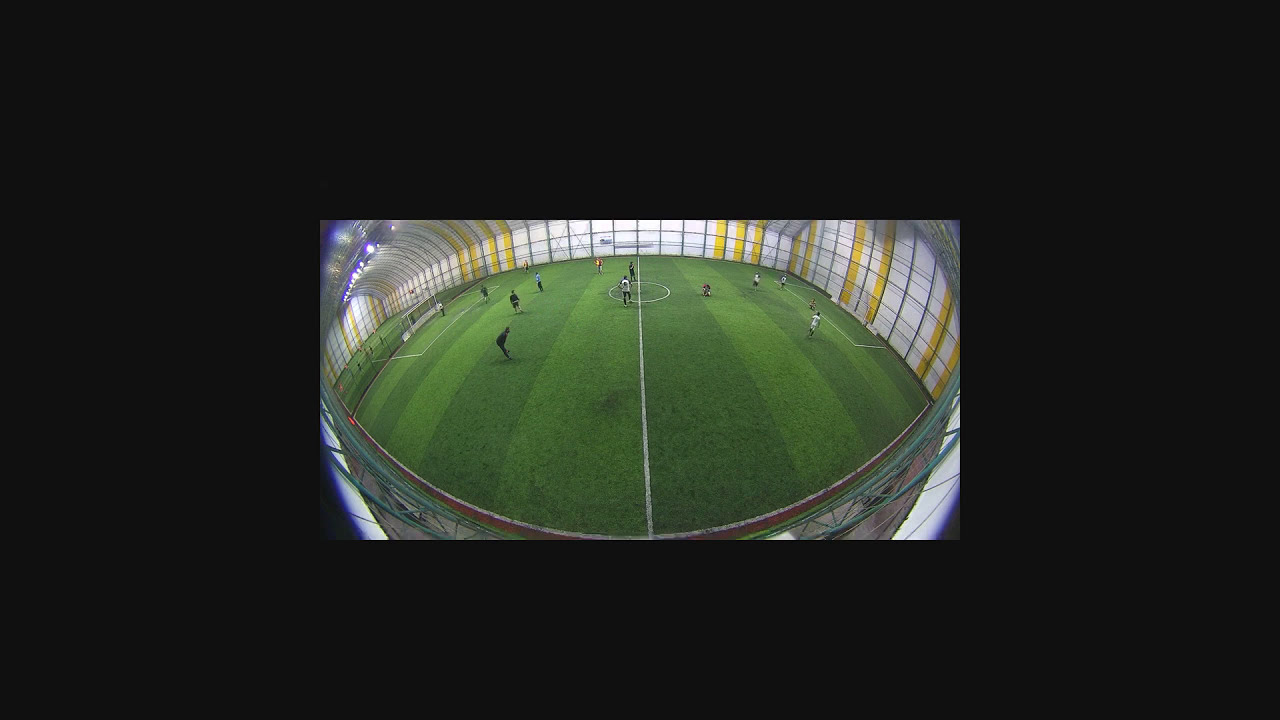The image captures an indoor soccer field viewed through a fishbowl lens, creating a wide-angle, spherical distortion. The field itself, depicted with alternating light and dark green grass stripes, features a central white line and a circle at the midfield. Players are seen positioned on either side of the center line, with three in white uniforms on the right, one red-clad player near the center, alongside others in black, blue, and red uniforms spread across different areas. Each side of the pitch has a goal post with white nets, and rectangular boundary markings clearly visible. The indoor venue is distinguished by its bright, transparent, white walls adorned with yellow stripes and black vertical lines, supported by metal framing in green. Additionally, overhead lighting illuminates the scene. The entire image is framed with a thick black border, enhancing the focus on the field below. In the bottom left corner of the image, another soccer pitch is faintly visible, suggesting a multi-purpose sports facility.